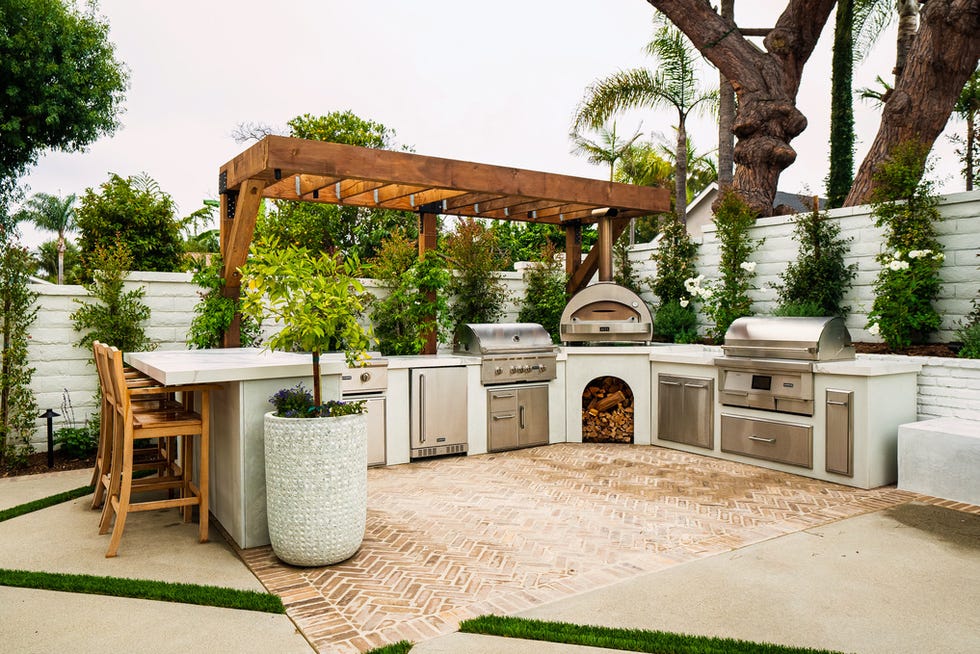This image depicts a detailed and expansive outdoor barbecue area located in a backyard, showcasing an impressive array of grilling and cooking equipment. The central highlight is a built-in barbecuing grill nestled within a brown brick cooking area. Adjacent to this, there's a small furnace packed with firewood and an overhead grill. The kitchen setup also includes a pressure cooker, a silver and metallic oven, a fridge, and several drawers, all adding to the sleek, functional design.

On the left side, an island table with a marble countertop is accompanied by several bar stools neatly tucked in. This countertop table seamlessly blends functionality and style, creating a perfect spot for social gatherings. The surrounding area features a patchwork of concrete with grass growing in artistic patterns, enhancing the aesthetic appeal.

Above the barbecue area, there’s a wooden structure, possibly serving an ornamental purpose. The outdoor space is encircled by lush greenery, including a couple of palm trees and other large oak trees, contributing to the tropical ambiance. Additional details include a tall white fence that runs along the perimeter, behind which more trees are visible. A large pot with a small tree is placed near the left area, adding a touch of nature.

In the distance, the top of another house peeks from the right corner, underlining the residential setting, while the sunny sky above completes the vibrant backyard scene.